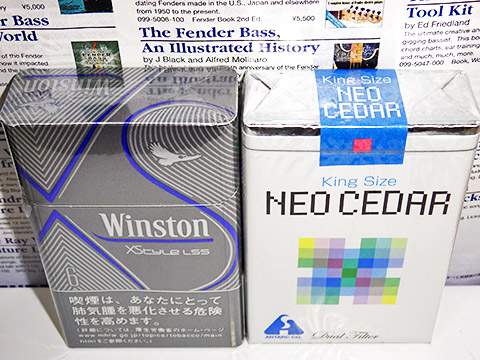The image displays an overhead view of two cigarette packs positioned side by side on a colorful magazine page filled with various articles and posts. The pack on the left is a rectangular gray packet featuring the brand name "Winston" in blue letters, accompanied by a white flying bird logo. Below the brand name, there are Japanese characters, and it also says "XS." The right pack, also rectangular but primarily white, displays "Neo Cedar King Size" at the top in blue letters with a blue ribbon overlay. On the front, "Neo Cedar" is written in black, and "King Size" appears again in blue. This pack also has a logo consisting of a array of multicolored squares and an additional blue emblem in the bottom left corner. Both packs suggest a vibrant, commercial setting, emphasizing their distinct branding against the backdrop of varied printed materials.